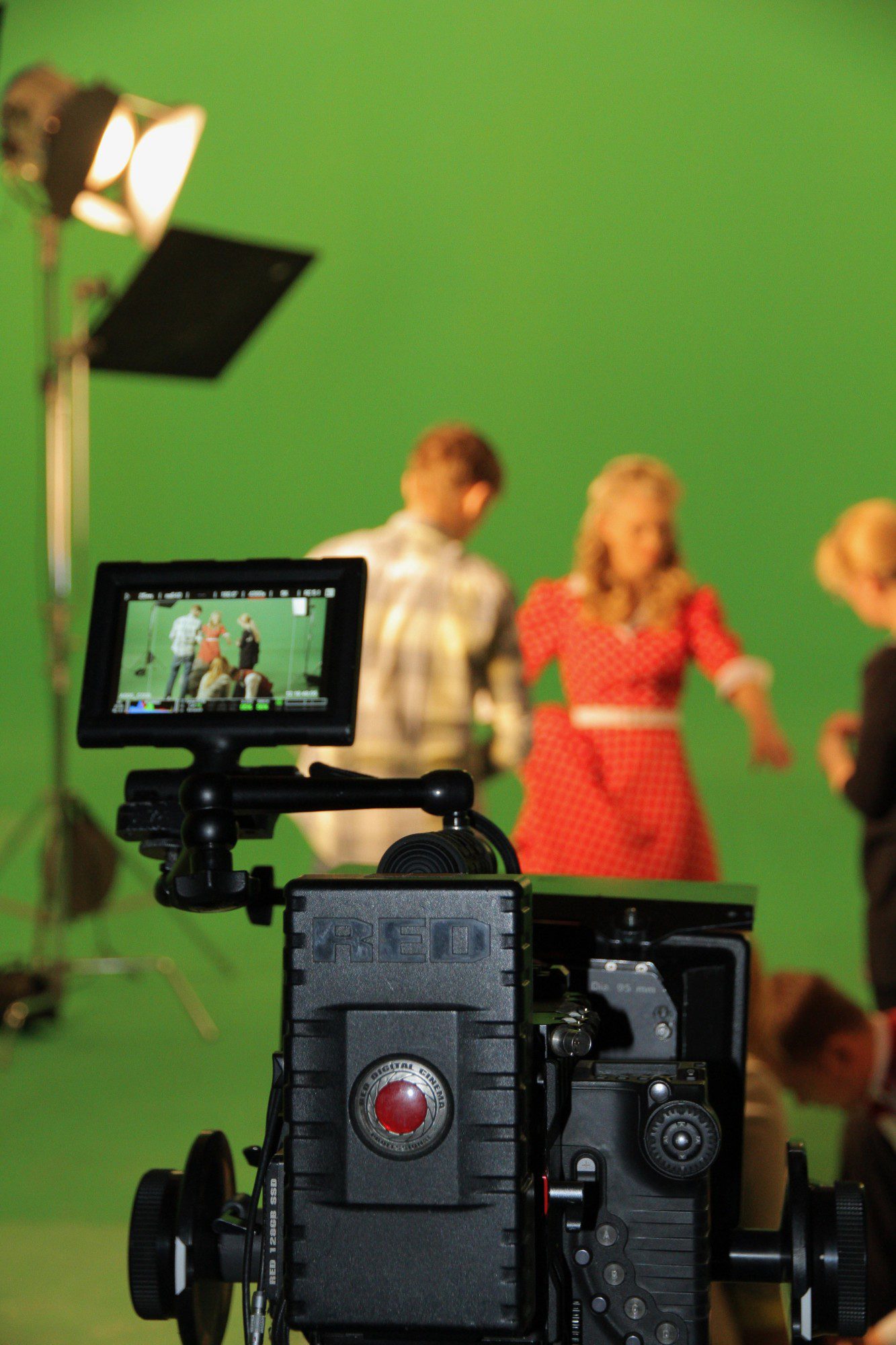This full-color, vertically rectangular indoor photograph, taken under artificial light, features a film set with a vivid green screen backdrop. Central to the image is a professional film camera, predominantly black with a red digital display and a screen showing what the camera captures. The camera is positioned at the bottom center, with its base closer to the viewer and its screen slightly elevated to the left. In the upper left corner, professional stage lighting illuminates the scene, casting shadows on the green screen backdrop.

Three individuals are prominently featured, albeit slightly out of focus. At the center, a woman with long blonde hair, wearing a red dress adorned with a white belt and sleeve cuffs, face forward. To her right, a second woman with blonde hair in a dark outfit observes her, depicted in a side profile. On the left side, a man with short hair dressed in a plaid shirt stands with his back to the viewer. Additionally, in the lower right corner, a fourth person with brown hair, partially obscured and bending down, is barely visible. The collaborative efforts of these individuals, combined with the sophisticated equipment and setting, emphasize the behind-the-scenes workings of a professional film shoot.